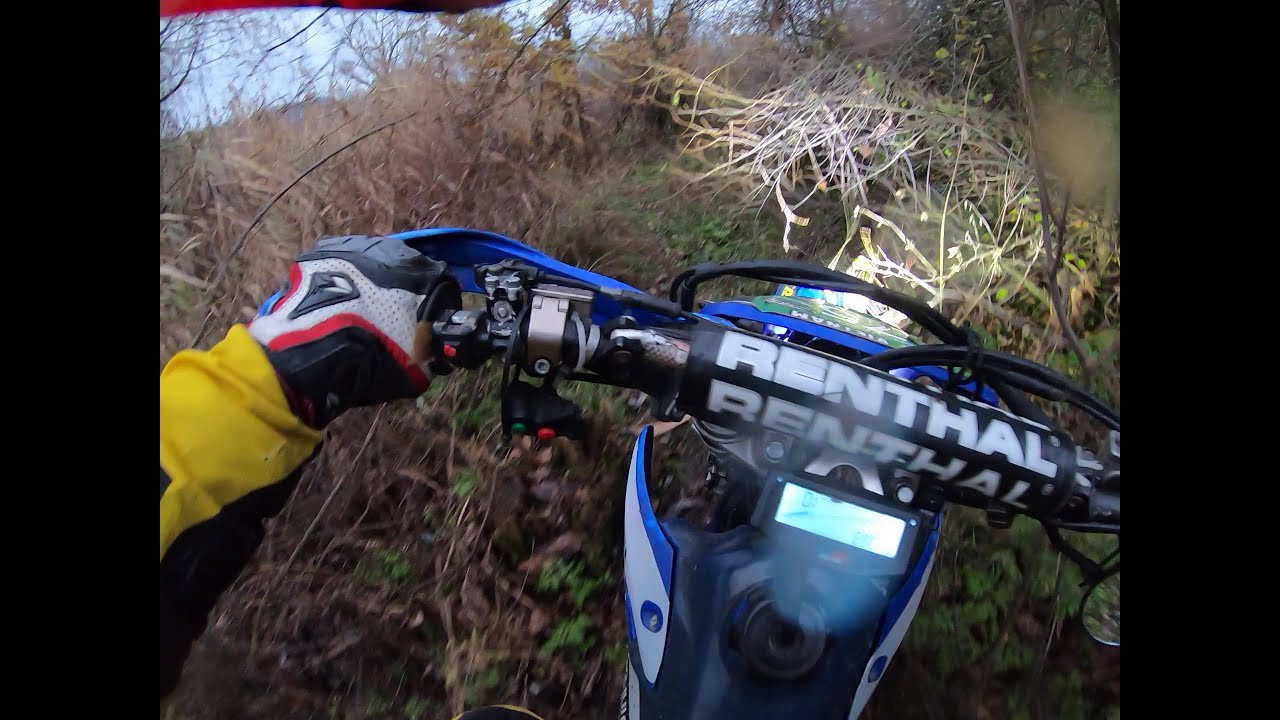The image is a point-of-view shot from a rider navigating a blue dirt bike with a main frame featuring blue and white stripes. The bike is moving through a thick, brushy area filled with twigs, branches, shrubs, and brambles in a wooded environment, with no visible path. Prominently displayed on the handlebar frame is padding branded 'Renthal' in large, bold, white, capitalized letters. The rider, dressed in a yellow and black motocross suit, and wearing black, white, and red gloves, is gripping the handlebars while their front light shines ahead despite the bright daylight. The image also features black vertical bars on the left and right sides.